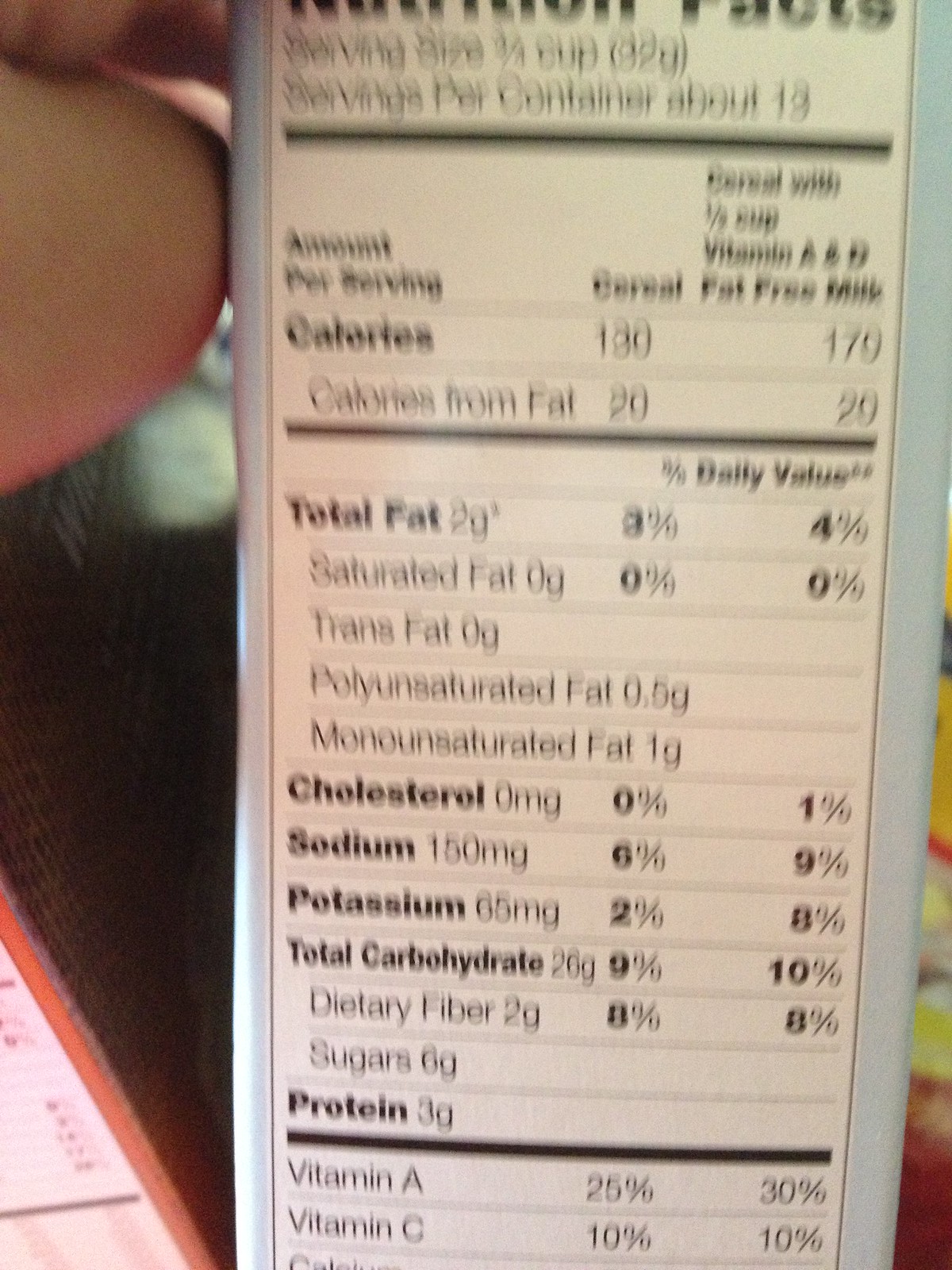The image features a nutrition label on the side of a box, slightly out of focus. The label belongs to "Mount Perseverance Cereal" and provides nutritional information for a serving size of three-fourths of a cup. The label itself is vertically rectangular, with a white background and black text. There is also a light blue border that frames the label. A person's fingers, which appear to be white, are partially visible touching the box. In the background, another box with an orange label is lying down, suggesting that the individual might be taking multiple photos of different product boxes.